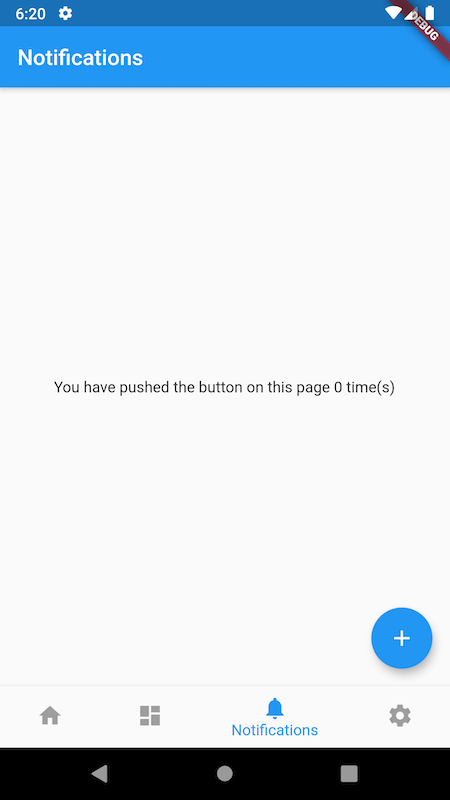This screenshot displays the user interface of a mobile phone app in a vertical aspect ratio, suggesting it was captured from a smartphone. At the very top, the phone's status bar is visible, showing essential indicators like the time, battery power level, and Wi-Fi signal strength. Immediately below, there is a blue notification banner with white text, which currently states that there are no notifications set up or labeled.

The main part of the screen is largely occupied by a gray background, emphasizing the absence of notifications. In contrast, the bottom right corner features a prominent circular icon with a plus sign, signifying the option to add a new notification.

At the very bottom of the app interface, there is a navigation bar with several icons: a home icon, a multi-square icon, a bell icon, and a cogwheel icon, providing quick access to different features of the app. Beneath this UI menu, the phone's default navigation bar is displayed, including the back button, home button, and an option to close all apps.